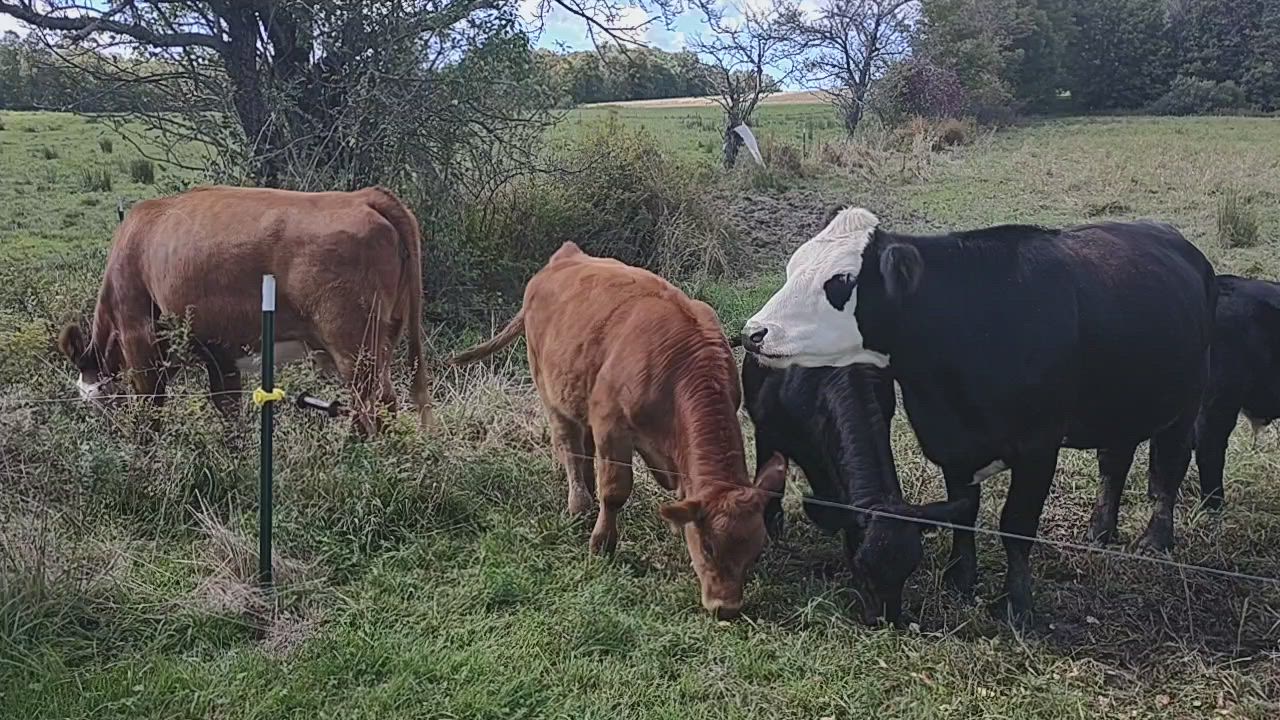In this vibrant outdoor photograph, five distinct cows are seen grazing in a lush, grassy field. Dominating the scene, a serene blue sky, dotted with numerous white clouds, stretches across the upper center, tapering into big, lush green trees on the right, indicating a thick forest in the distance. The tree line extends across the background, providing a picturesque natural frame.

Occupying the left side of the image, a large brown cow stands with its side to the camera, head down, and tail hanging behind. Just to the right, another brown cow also has its head lowered towards the grass, with its tail slightly angled to the left. Next to them, a small, jet-black cow, possibly a calf, is seen reaching down to graze.

Adjacent to the calf, a prominent large cow, likely its mother, displays a striking appearance with a black body, white face, and black patches around its eyes and nose. This cow is in profile, looking to the left. Partially visible on the far right, the hindquarters of another black cow are captured. In the foreground, an electric fence, comprising a thin metal wire supported by a green pole, stretches across the scene from left to right, providing a subtle barrier between the cows and the camera.

Enhancing the composition, a large tree on the left, just behind the first brown cow, and a dense bush to its right contribute additional texture and depth to this pastoral landscape.